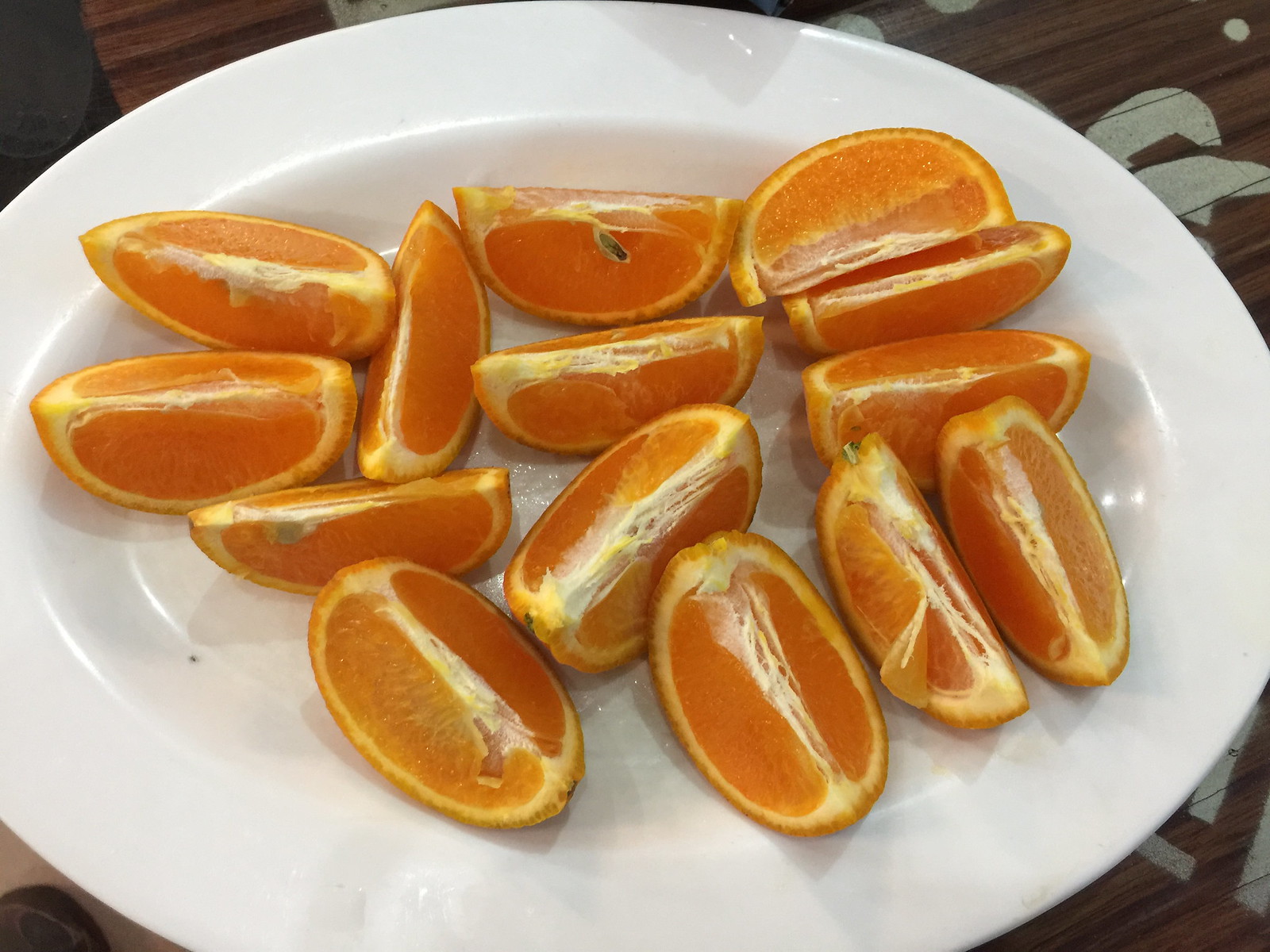The image is a color photograph taken from a top-down, 45-degree angle, showcasing a large, white, oval ceramic dish with a pronounced edge and a central dip, resembling a soup bowl. This dish is scattered with approximately 15 vibrant orange wedges arranged haphazardly, with the bright flesh facing up and the rind down. Some of the wedges display visible pith and seeds, adding to their natural appearance. The background reveals portions of a dark wooden surface, partially obscured by the plate, with indistinct imprinting visible on the wood. The overall presentation suggests a scene of juicy, freshly cut oranges ready to be enjoyed.